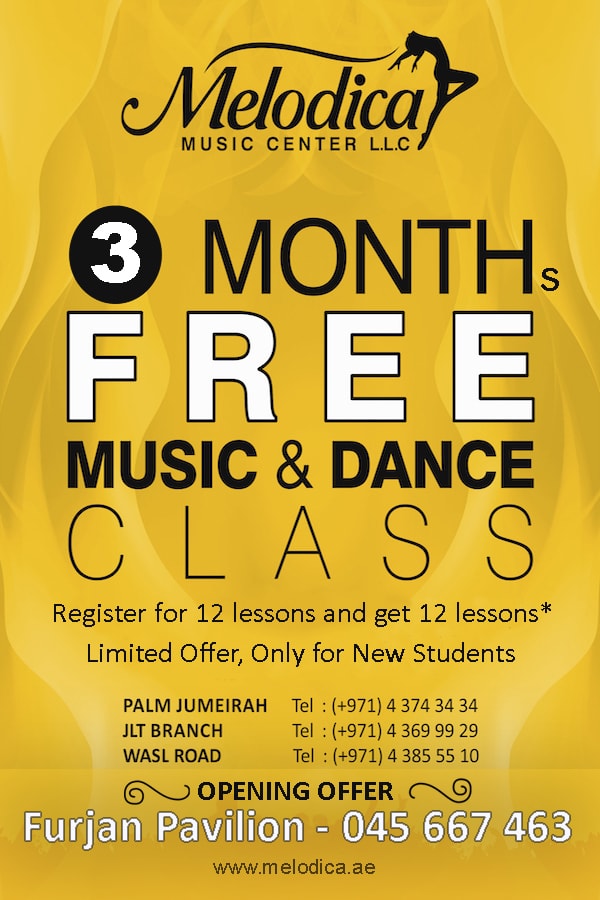The flyer is rectangular-shaped and approximately twice as tall as it is wide. The background is a yellowish-gold color with the faint outline of two hands extending upward from the bottom, appearing to make a palm motion.

At the top, there is a thin black line that extends upward and then to the right. At the tip of this line, there is a silhouette of a woman in a pose reminiscent of the iconic "Flashdance" scene, leaning back with her hands outstretched to the left.

Below the line, in large black lettering, the flyer boldly displays "MELODICA," followed by "Music Center LLC" in smaller, all-capital letters.

Towards the lower left, there is a black circle with a large bold red "3". Next to it, "MONTH" is written in large, all-capital, black letters with a small "s" at the end. Beneath that, the word "FREE" is prominently displayed in bolded white text with a black border.

Further down, in large, bold black letters, the flyer advertises "Music and Dance Class." Below this, in normal black font, it states, "Register for 12 lessons and get 12 lessons" with an asterisk pointing to "limited offer, only for new students."

At the bottom of the flyer, there are contact details for three locations with corresponding telephone numbers: Palm Jumeirah, JLT Branch, and WASL Road. The phrase "Opening Offer" is noted with a decorative line running alongside it.

Across the bottom, the flyer mentions "For Jam Pavilion" with a phone number listed. Finally, in small black lettering at the very bottom, the website is displayed: www.melodica.ie.